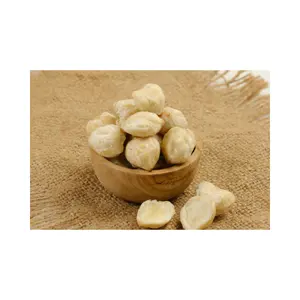The image depicts a light brown, wooden bowl resting on a tan, straw-like rug that is slightly frayed at the upper right-hand corner. Inside the bowl, there are several circular or oval-shaped edible items that are light yellowish-white in color, resembling either nuts, peanuts, or possibly small pieces of bread. These edible pieces are piled high, forming a pyramid-like structure, with one prominent piece at the top. Additionally, three of these pieces are placed outside the bowl on the rug, contributing to the overall count of approximately seven or eight visible pieces. The simple composition highlights the organic textures and neutral tones of both the bowl and its surroundings.